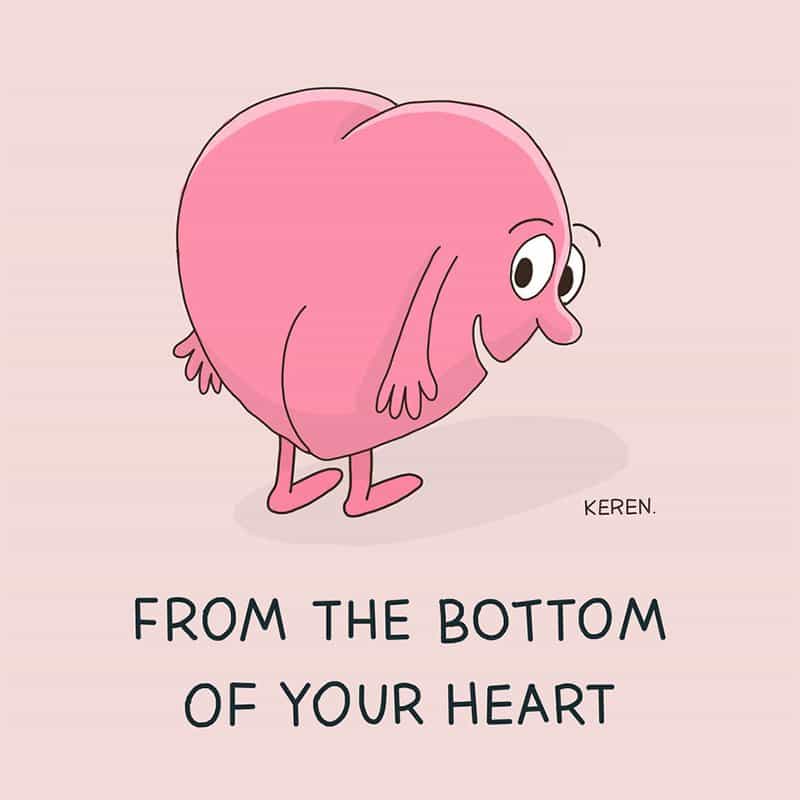The humorous cartoon image features a stylized pink heart with a faint pink background. The heart, facing away but turning to look at us, has big, white cartoonish eyes, a protruding nose, a wide smile, and expressive eyebrows that make it appear surprised. It also has arms with hands and feet. Notably, the backside of the heart, including its butt crack, is visible. Below the heart, a shadow slightly darker than the background is cast. At the bottom of the image, the caption reads "FROM THE BOTTOM OF YOUR HEART" in all caps. Just above this text, the name "K-E-R-E-N" is inscribed, likely indicating the illustrator.